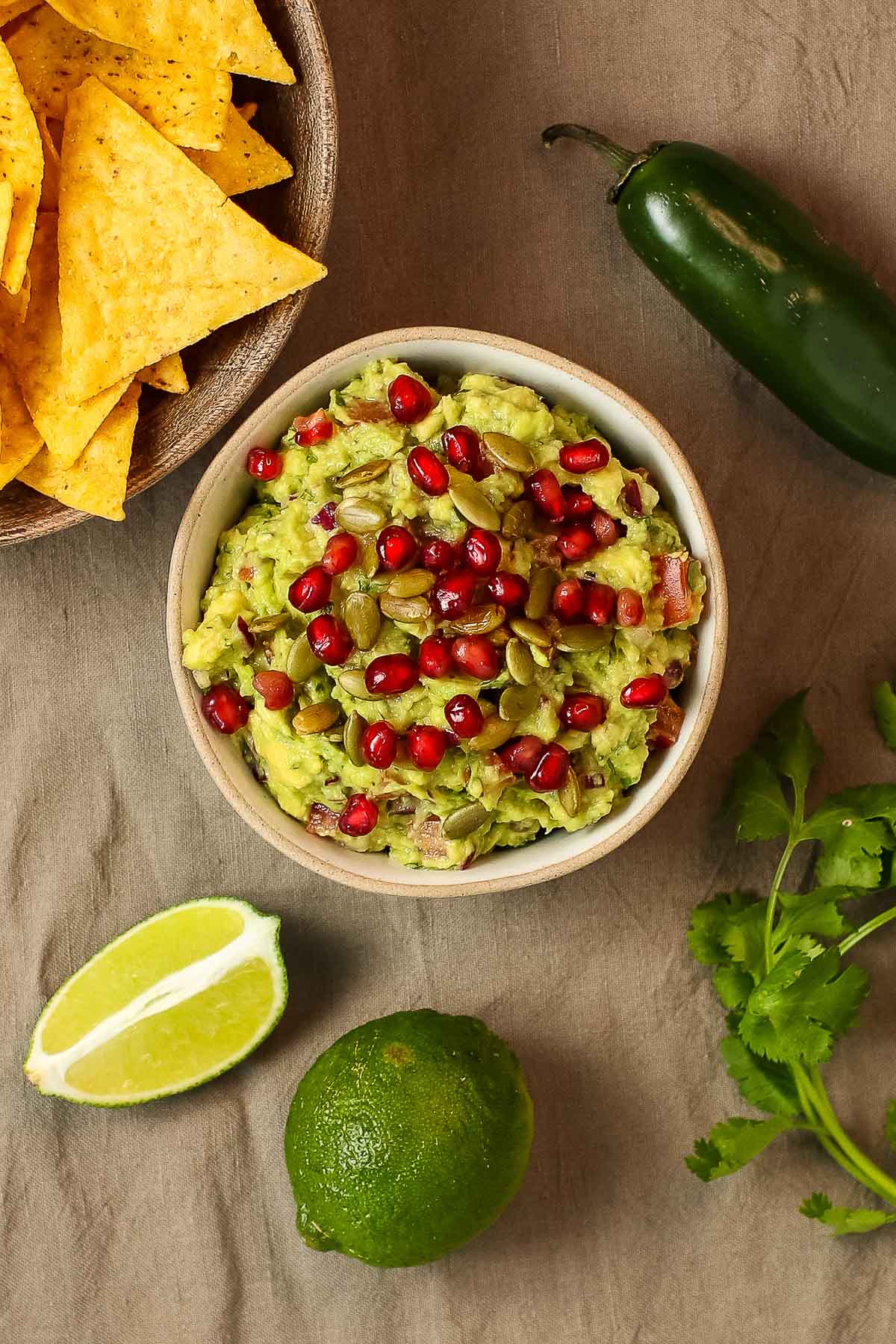In this detailed and vibrant close-up photo, a brown circular bowl brimming with fresh guacamole takes center stage. The guacamole is a lively green with pomegranate seeds and what appears to be an assortment of sunflower and pistachio seeds sprinkled throughout. There are noticeable chunks of avocado, tomato, and onion mixed in, enhancing its texture and freshness. To the left of the guacamole, a larger brown bowl filled with orange tortilla chips is partially visible. Below the guacamole, a whole lime and a lime wedge are arranged together, adding a zesty touch to the composition. On the right side of the image, a sprig of fresh cilantro rests beside a green chili pepper, adding pops of vibrant green. The scene is set against a rich brown tablecloth, which provides a warm and earthy backdrop to the colorful and appetizing spread. The photo beautifully captures the freshness and detailed preparation of the guacamole and its accompaniments, with just the edges of the tortilla chip bowl, the chili pepper, and cilantro visible, framing the guacamole in the center.